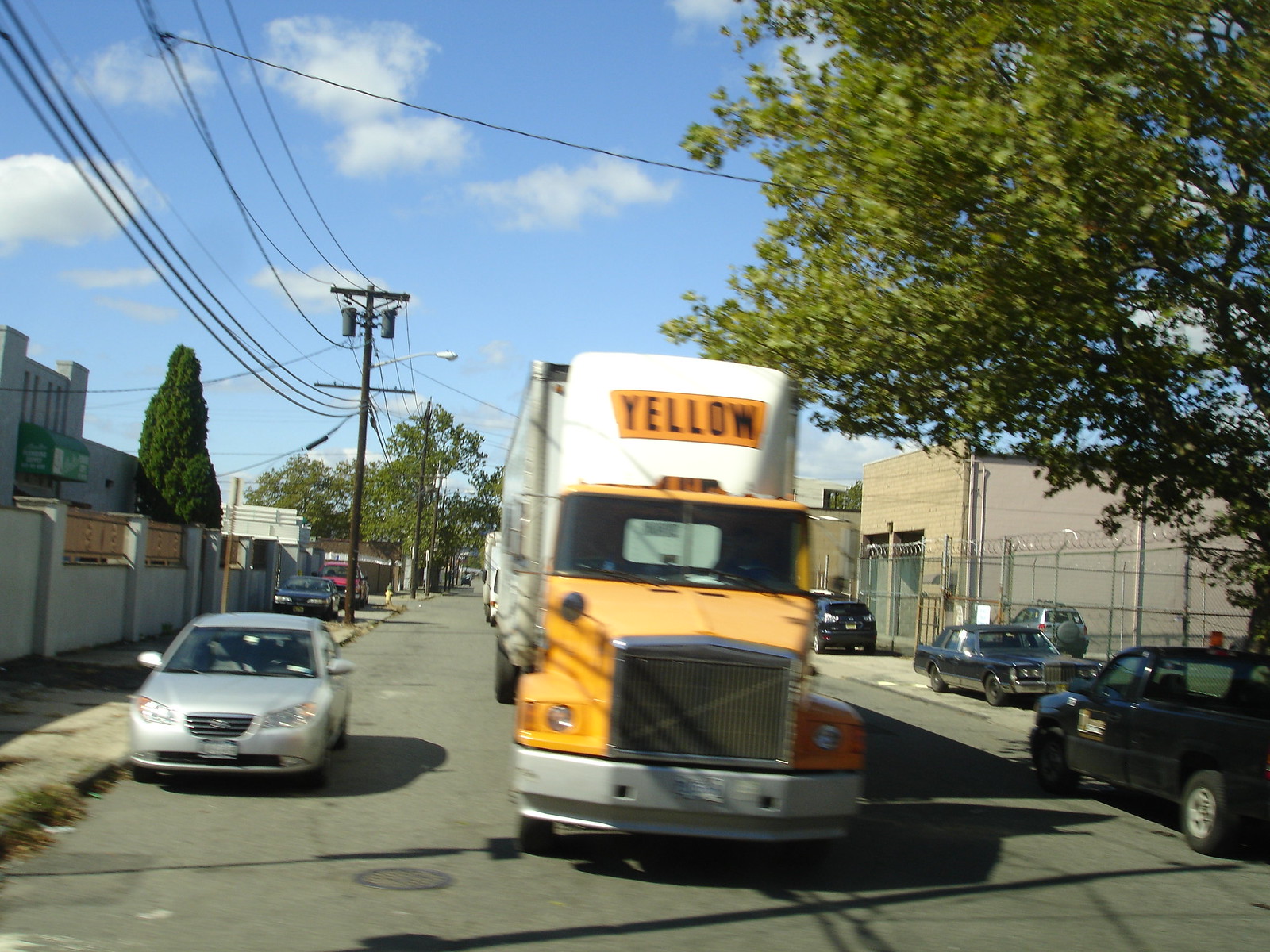A vibrant yellow semi-truck with a white trailer, marked with the word "yellow" in bold black letters inside a yellow square on the top of the trailer, is prominently featured. To the left of the semi-truck is a sleek silver car. On the right side, there is a succession of vehicles: a black truck, followed by three black cars, all parked behind a chain-link fence. Another black car is visible to the left in the background, along with a red car nearby. The scene is interspersed with multiple power lines and poles, stretching horizontally and vertically across the image.

To the right of the scene, lush green trees provide a natural backdrop. More trees along with a wall and buildings can be seen to the left. Additionally, there is a building on the right side. The street, colored in a dull gray, has a distinct circular marking on the front left. The sky hangs above in a serene blue with scattered white clouds, while a street light stands at the middle left of the scene, adding to the urban ambiance.